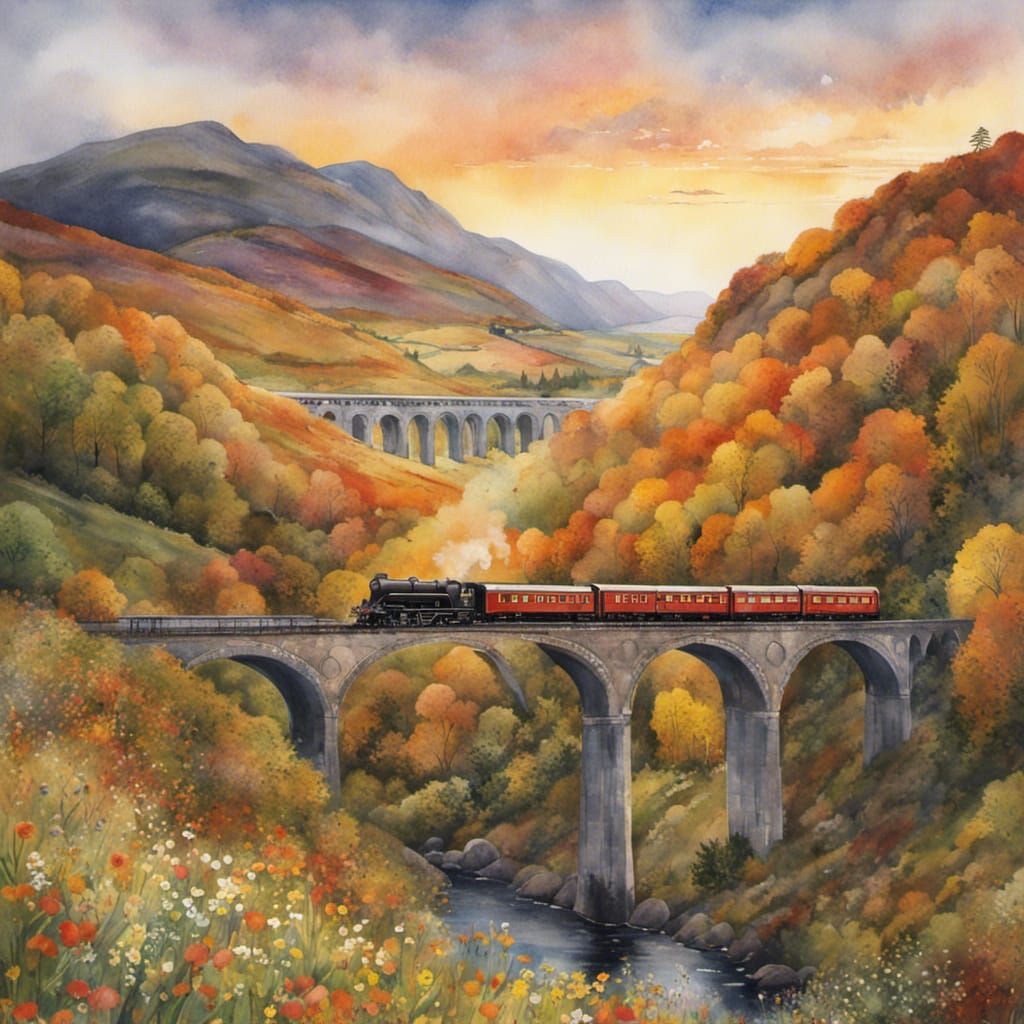This is an intricate painting with no border, depicting a picturesque landscape in autumn. The sky at the top is mostly cloudy with feathery white clouds tinged with light orange and yellow, with small slivers of blue visible. A range of mountains occupies the upper left, blending medium and dark browns with some touches of blue, gray, tan, and reddish hues. Descending from the mountains, the landscape transitions into lush, forested hills that exhibit vibrant autumn colors, including shades of green, orange, yellow, and some light reddish tones.

Dominating the center, a grand brownstone bridge with large arch cutouts spans a narrow body of water, which is a clear, calm lake bordered by gray stones. A black engine with five red cars, marked by yellow around the windows, traverses this bridge. In the far background, another stone bridge is visible, further enhancing the depth of the scene. Above these elements, a small town or large home can be distinguished, draped in the distance under the sumptuous sky.

The foreground is lively with wildflowers in various colors including white, red, yellow, and orange, framing the left hill and spreading towards the bottom right corner. This complex and vivid depiction illustrates not only the change of seasons but also the harmonious interplay of natural elements and human engineering.